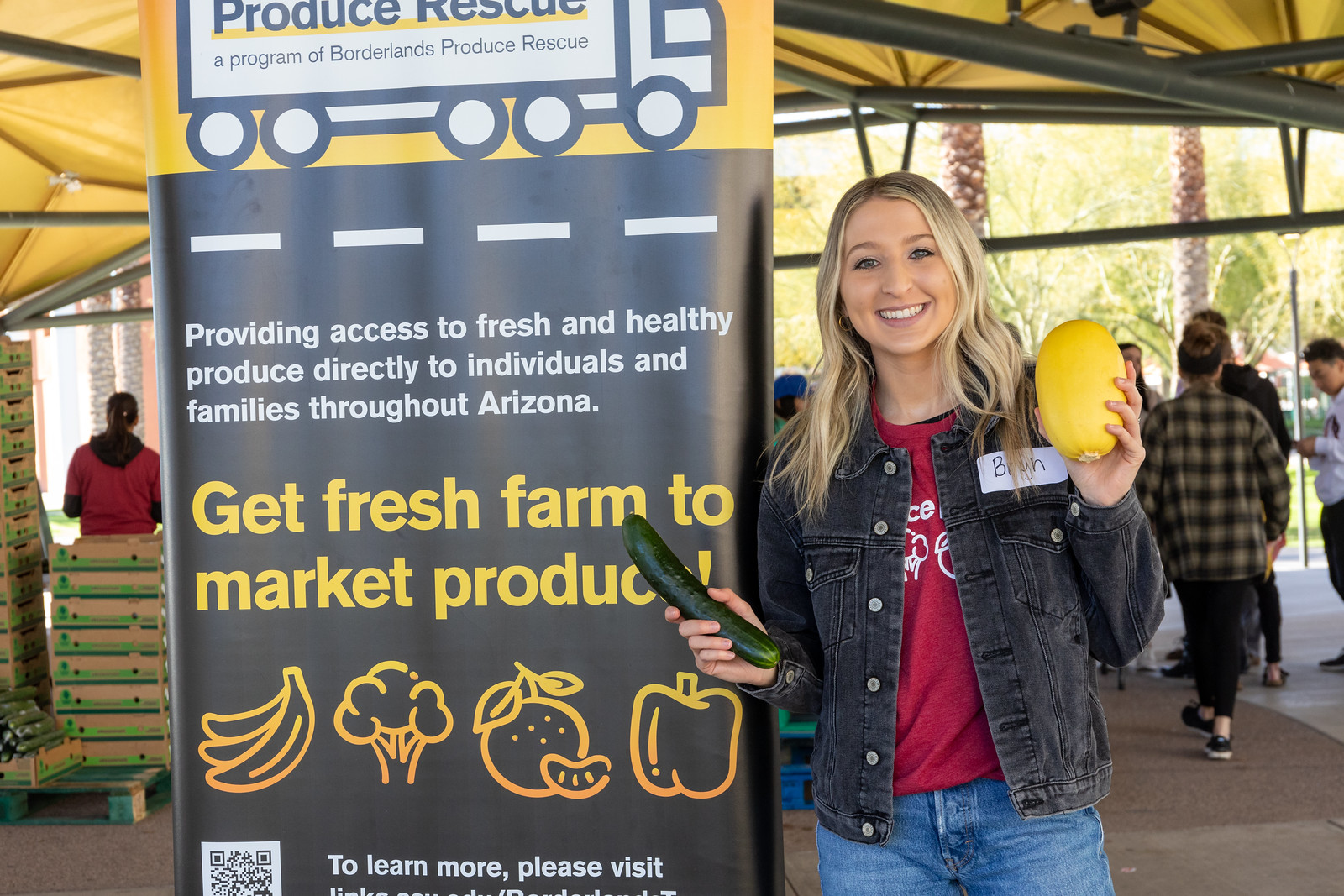In a bustling setting reminiscent of a farmer's market, a woman with shoulder-length blonde hair and a warm smile is the focus of the photograph. Dressed in a black jean jacket with a small handwritten name tag, a red t-shirt, and blue jeans, she stands confidently holding a large yellow fruit in her left hand, possibly a mango or grapefruit, alongside a green cucumber in her right hand. Behind her, an animated crowd and pallets of fresh produce set a lively backdrop. Beside her, a prominent banner catches the eye with its vibrant yellow top featuring an illustration of a truck with five wheels and blue text that reads “Produce Rescue, a program of Borderlands Produce Rescue.” The rest of the banner has a black background with the message “providing access to fresh and healthy produce directly to individuals and families through Arizona" in white text, followed by bold yellow text stating “Get Fresh Farm to Market Produce.” At the bottom, cartoonish outlines of bananas, broccoli, an orange, and a bell pepper add a whimsical touch, concluding with an invitation to learn more via a QR code.